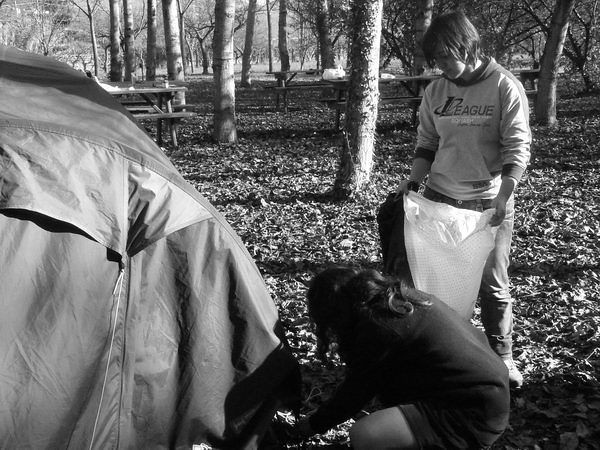In this black and white photograph, likely captured in the middle of the day, a picturesque park setting unfolds. The ground is lush with grass and scattered leaves, providing a natural base for the scene. In the center foreground, a woman is squatting near the ground, seemingly picking something up. To her right, another woman stands, holding a trash bag open, aiding in the clean-up effort. The left side of the image reveals the back of a dark tent, as well as the back of someone's coat. Within the background, picnic tables, some with bottles and containers on top, are dotted among the trees that stretch into the distance. This well-illuminated public space, characterized by wooden benches and the expansive woodland, conveys a serene and communal outdoor environment.